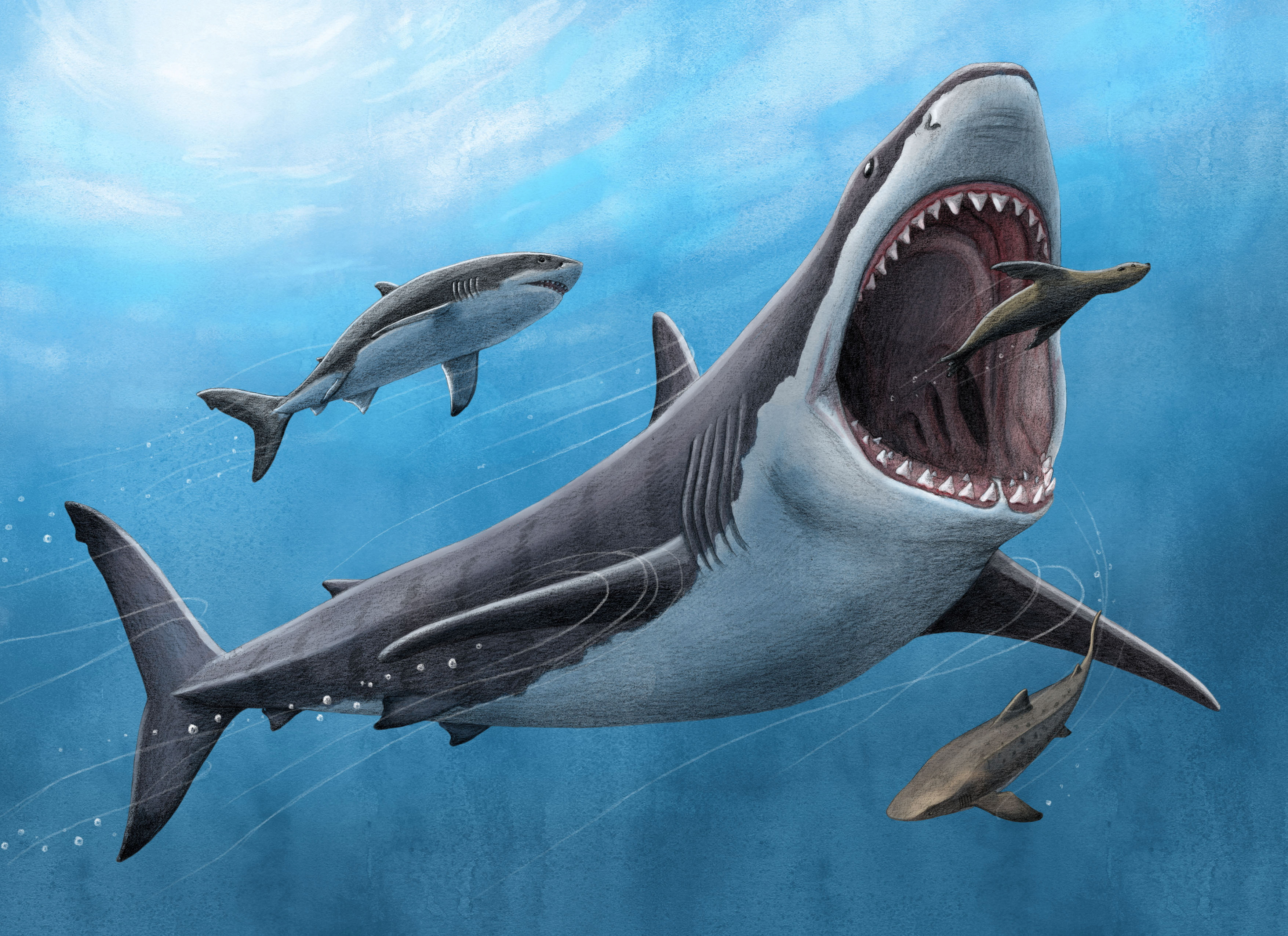This is a detailed, horizontally aligned rectangular painting of an underwater scene centered around a large gray-white shark, likely a tiger shark, with dark gray stripes. The shark, depicted with large fins and a gaping mouth full of sharp teeth, is positioned at a slight upward angle, with its tail in the lower left corner and its head in the upper right corner, about to devour a small brown sea otter. The background features swirling blue and white hues, especially pronounced in the upper left corner where sunlight breaks through the water's surface. Accompanying the main shark are two smaller sharks: one below it, resembling a miniature whale, and another above, both sharing the same silver and gray coloring and distinct markings. The overall composition vividly captures the dynamic and perilous aquatic environment.